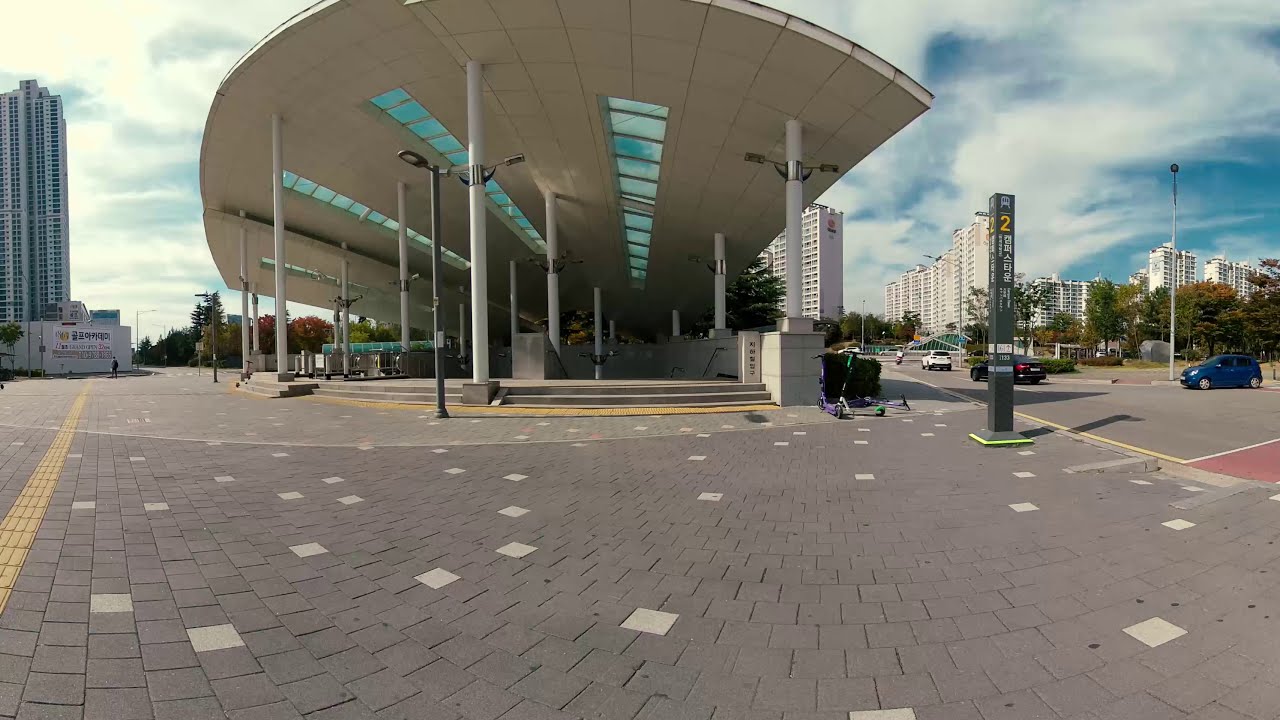This photograph captures a vibrant urban scene in an Asian city, showcasing a plaza that likely serves as a metro or bus station. The area is characterized by a large, curving roof with windows that let in daylight, creating a fish-eye lens effect. This roof covers an outdoor walking area paved with gray rectangular bricks interspersed with white bricks in a decorative pattern. Prominently featured is a tall post with the number "2" and Asian writing beneath it, suggesting it might be an entrance point to the underground station. To the left of the plaza, stands a white skyscraper, while the right side is lined with a series of other tall buildings, each featuring multiple levels. The sky above is a clear blue, dotted with whispering clouds, enhancing the bright and airy atmosphere of the station. In the distance, vehicles can be seen moving along a road adjacent to the plaza, integrating the scene seamlessly into the bustling cityscape.